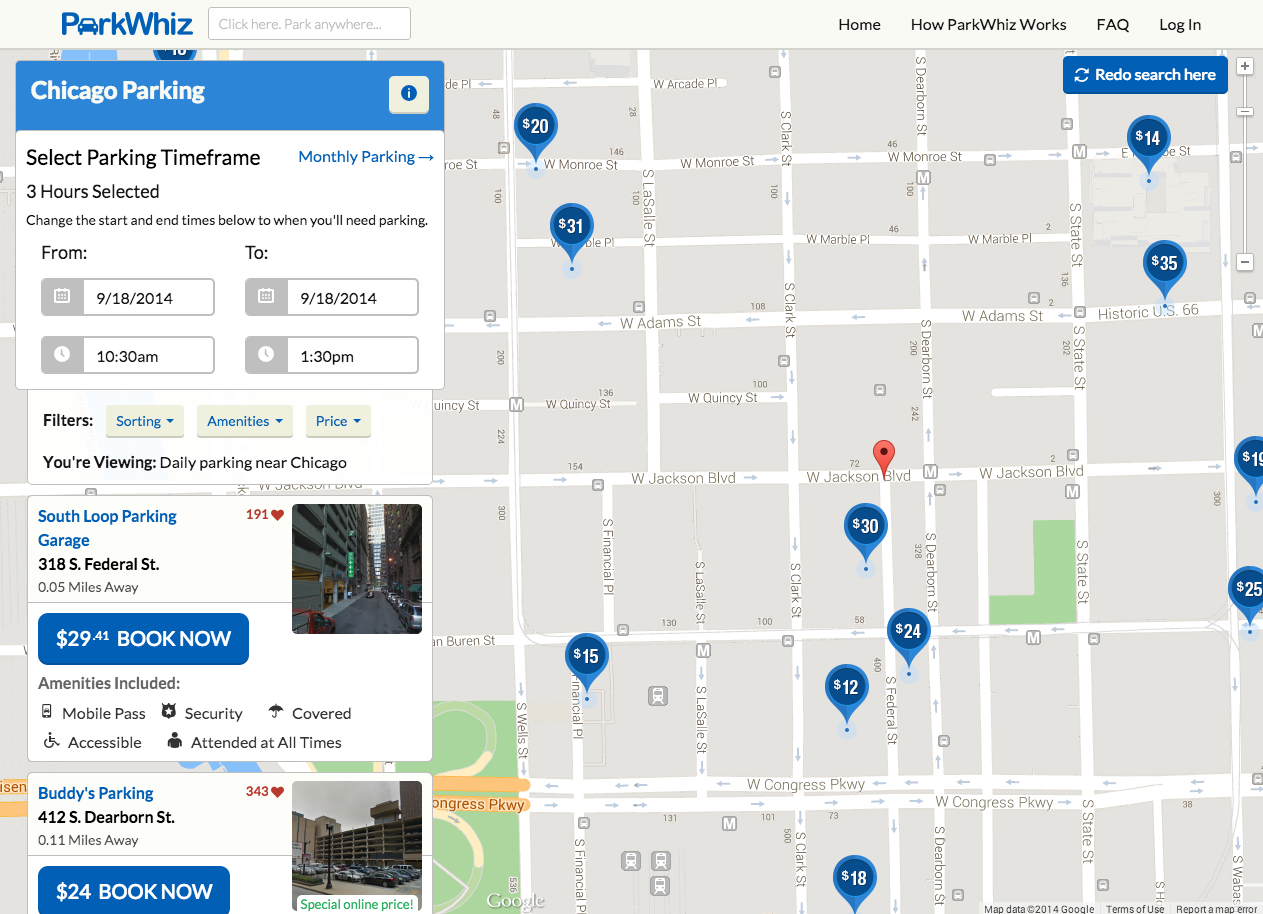This image is a detailed top-down screenshot of a map showing an area densely populated with blue pins, each representing a parking location. At the top-left corner, the header features the name of the company, "Park Wiz," with the 'A' stylized as a car icon in blue. Adjacent to the company name is a search box. On the top-right of the header, there are navigational options including "Home" with a drop-down menu, "How Park Wiz Works," "FAQ," and a "Login" button.

On the left side of the image, there is a vertical column containing various white information boxes. The top box features a blue header with the text "Chicago Parking" in white, followed by a section prompting users to "Select Parking Timeframe." This section includes four input boxes for entering the date and time for parking. Below this, there are two promotional ads for specific parking structures. Each ad displays a large blue rectangle with white text, showing the price and a "Book Now" button, with one ad offering parking for $29.41 and the other for $24.

The main body of the image is a grayscale map with green areas depicting land features and white lines indicating roads. Scattered across the map are numerous blue pins, each marking the location of different parking structures available for booking. The overall design is clean and organized, emphasizing the multitude of parking options available in the highlighted area.